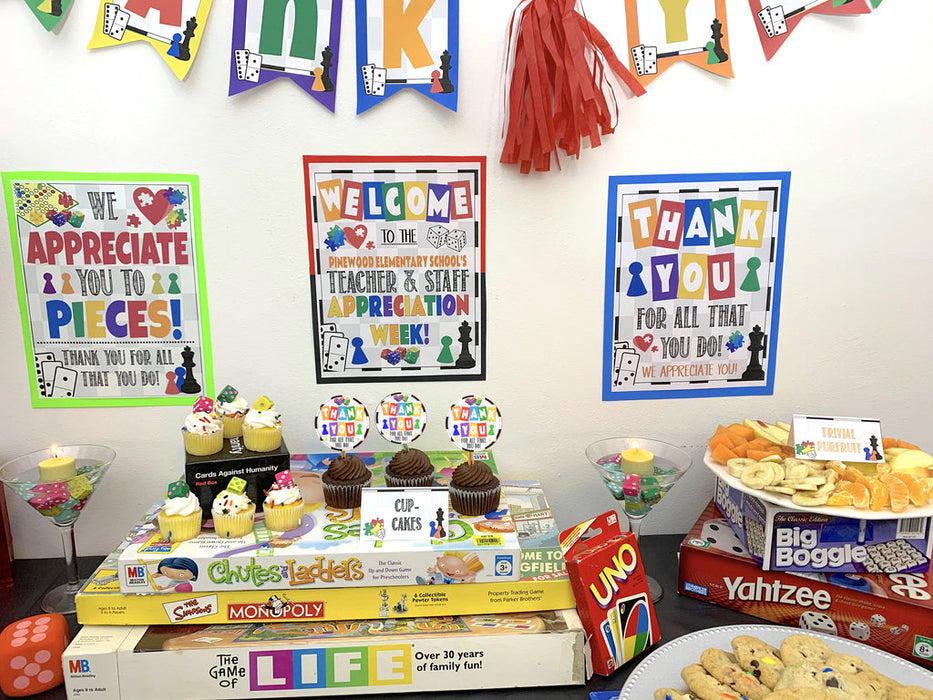The photograph captures a heartwarming scene from a special event, likely Teacher and Staff Appreciation Week at Pinewood Elementary School. A partially visible banner at the top of the image spells out "Thank You," with colorful red paper streamers hanging down, adding festivity to the setting.

Three posters are mounted on a pristine white wall. The leftmost poster reads, "We appreciate you to pieces. Thank you for all that you do," with the word "appreciate" highlighted in red and "pieces" in multiple colors. The centerpiece poster announces, "Welcome to the Pinewood Elementary School's Teacher and Staff Appreciation Week," with "Pinewood Elementary School" displayed in vibrant orange letters, while other text features a mix of black and various colors. The rightmost poster repeats the sentiment, "Thank you for all that you do. We appreciate you," adorned in a mix of colors as well.

In front of the posters stands a black table laden with a variety of snacks and treats, including an array of cupcakes, cookies, and fruits. Underneath the edible delights, a collection of board games such as Monopoly, Life, Yahtzee, and Uno are neatly arranged. On the right side of the table, a small white placard features a playful spin on the classic game "Trivial Pursuit," instead reading "Per Fruit," cleverly paired with a platter of fresh fruit.